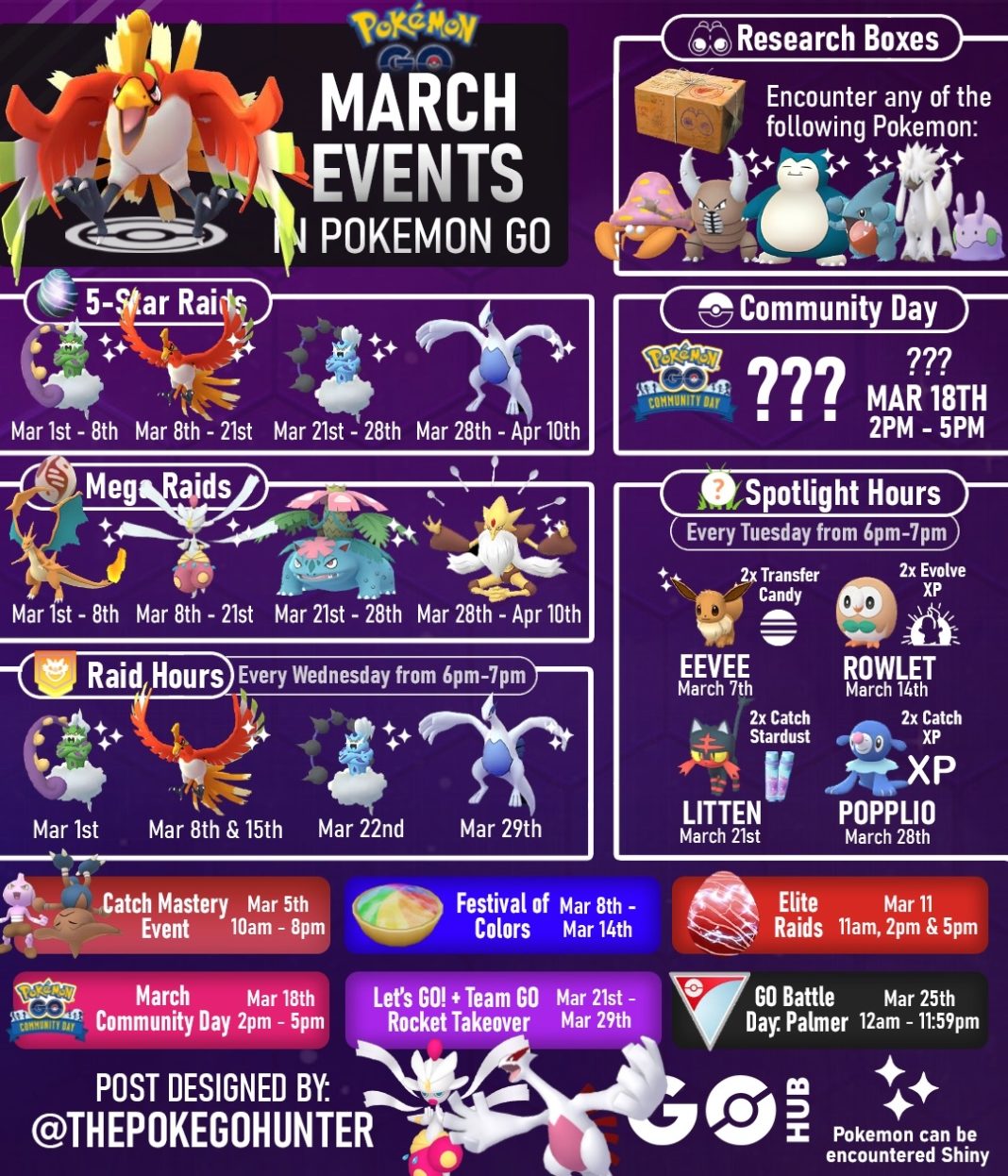In this detailed image, we see a vibrant and information-packed poster detailing the various events scheduled for March in Pokémon Go. 

At the top, the poster highlights "March Events," which include a wide array of activities and special occurrences throughout the month. Key events are meticulously listed with dates and times:
 
- **Research Boxes**: Offers encounters with various Pokémon.
- **5-Star Raids**: 
  - March 1st to 8th
  - March 8th to 21st
  - March 21st to 28th
  - March 28th to April 10th
  
- **Community Day**: Scheduled for March 18th, running from 2 PM to 5 PM.
- **Mega Raids**: Specific Pokémon available for capture in these unique raid battles.
- **Raid Hours**: Happening from 6 PM to 7 PM, a chance for more frequent raid encounters.

Additional Special Events:
- **Couch Mastery Events**: Taking place on March 5th from 10 AM to 8 PM, suggesting a day full of at-home activities.
- **Festival of Colors**: Celebrated from March 8th to March 14th.
- **Lights Raid**: On March 11th, from 11 AM to 2 PM and then again at 5 PM.
- **Let's Go Plus Team Go**: Event activities and encounters on March 21st.
- **Rocket Takeover**: Featuring Team Go Rocket battles.
- **Go Battle**: Special challenges and rewards tied to competitive play.

The poster is vividly designed to catch the eye, ensuring trainers do not miss any of these exciting opportunities to engage with the game throughout March.